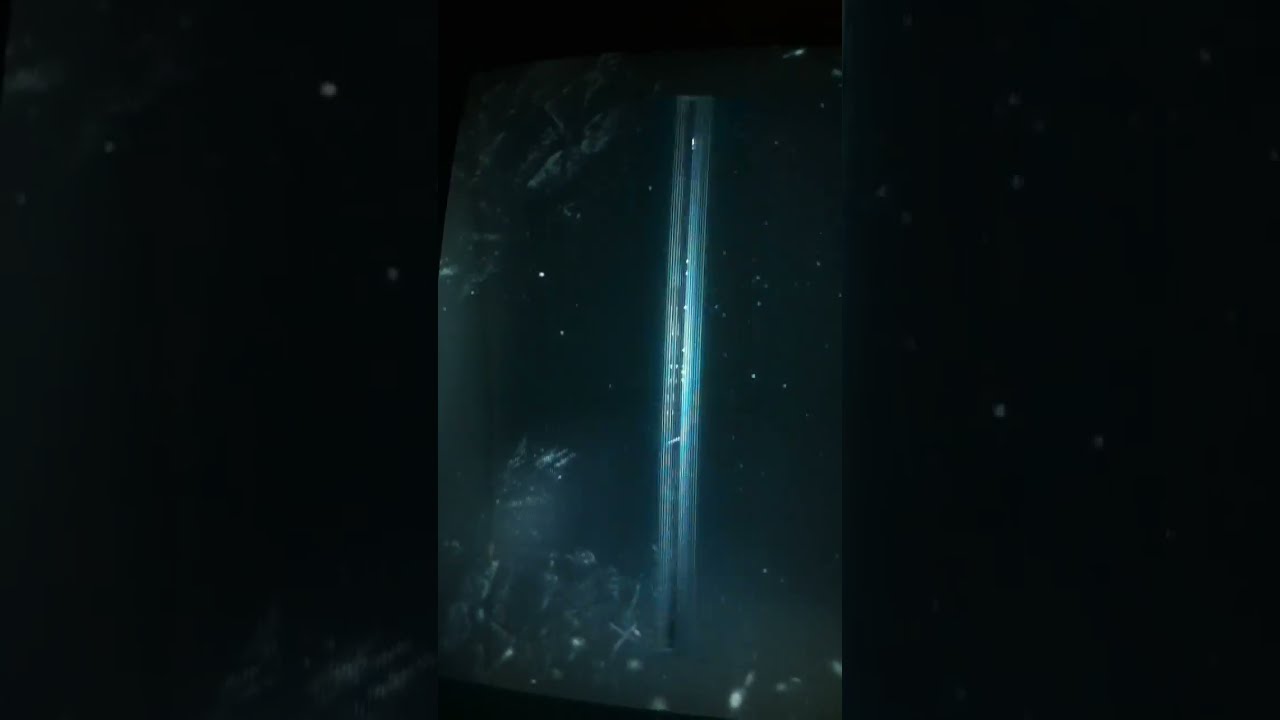This image is a dimly lit photograph with a distinctively digital appearance, captured seemingly as a screen shot or photograph of a monitor, positioned sideways. The central portion of the image is framed by two thick, black vertical panels, which dominate the left and right sides of the composition. The main focus of the image is a gray status bar exhibiting black text, apparently from a video game. 

The most legible part of the text includes "NHL 09" indicating a hockey game, alongside statuses like "Playing Offline" and "Away". Among the usernames visible are WATER (spelled W-A-T-E-V-A), possibly referencing a user, and others including Alan Erdman, John Watoya, and Blackout670. There also appears to be a green streak across the gray footer, adding a slight variation in color to the otherwise monochromatic palette. The text and details become more challenging to read towards the top part of the image.